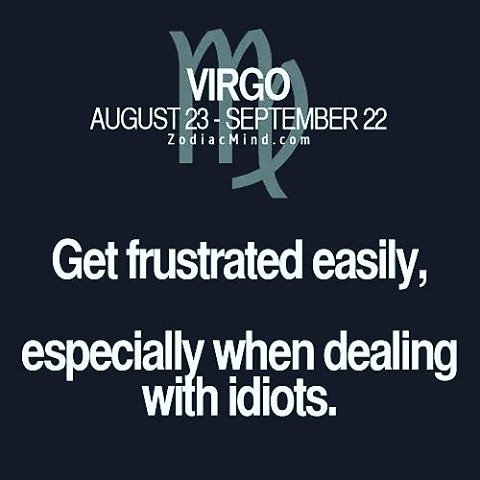The image features a promotional depiction of the Virgo zodiac sign. The background is a dark blue or pitch-black color, providing a stark contrast to the white text prominently displayed. At the top, the word "Virgo" is visible, followed by the dates "August 23rd - September 22nd." Below these dates, the text continues to emphasize Virgo traits, reading "Get frustrated easily, especially when dealing with idiots." This descriptive message is highly noticeable. At the bottom, the website "zodiacmind.com" is mentioned. Furthermore, a design element resembling an "M" pattern, which is not the traditional Virgo symbol, is placed at the top center of the image in a dark teal or dusty green hue. The overall layout and messaging make it clear that this square image is dedicated to explaining the Virgo zodiac sign.